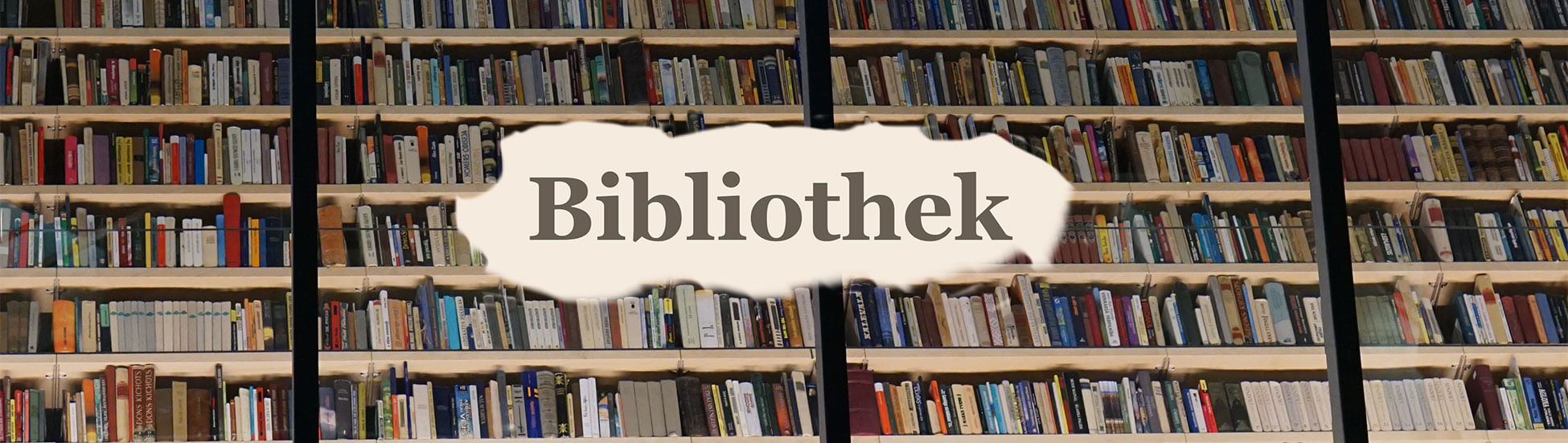The image showcases a library with a vast array of shelves filled with books of numerous colors, shapes, and sizes, giving an impression of up to a thousand books. The photo is wide but not very tall and captures four distinct sections of bookshelves, each containing approximately six shelves. These sections are divided by three black pillars, with one pillar centrally located and two others dividing the remaining space symmetrically. The image is taken from a low and tilted angle, thus showing the bottom of each shelf. The overall lighting is dim, except for the areas illuminated by the camera's flash. In the middle of the image, there is an overlaid, irregularly-shaped tan blob, possibly added through Photoshop. This blob features the word "Bibliothek" in dark gray letters, the German term for library, making the image appear as though it was marked or signed digitally rather than being part of the original photograph. The angles and the composition suggest a scene rich with literary treasures awaiting exploration.